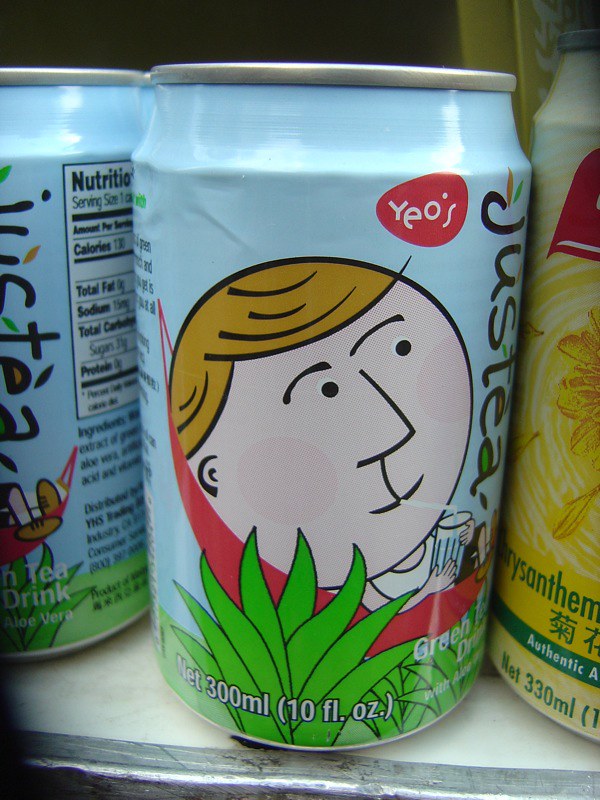A detailed close-up image captures a light blue beverage can standing on a white shelf with a metal front lip. The image is in portrait orientation. The can displays a whimsical, cartoony illustration featuring a large, circular human head with light-colored skin and yellow hair. The head has simple facial features and is turned upwards to the right. Just below the head, a small body in a white t-shirt is depicted lounging on a red chair that appears as a swoosh beneath the head. Green leaves ascend towards the head, adding a touch of nature to the design.

A pair of tiny arms protrude from the body, holding a glass with a beverage and a straw extending into the head’s mouth. The head is disproportionately large compared to the small torso and glass. At the top right corner of the can, a red egg-shaped label with white lettering spells out "Yeo's," and vertically down the right side, black lettering reads "JUSTEA." At the bottom of the can, white text indicates the volume: "Net 300 milliliters, 10 fluid ounces."

On the left edge of the shelf, part of another identical can is visible, showing partial nutrition facts. To the right, a glimpse of a yellow container can be seen.